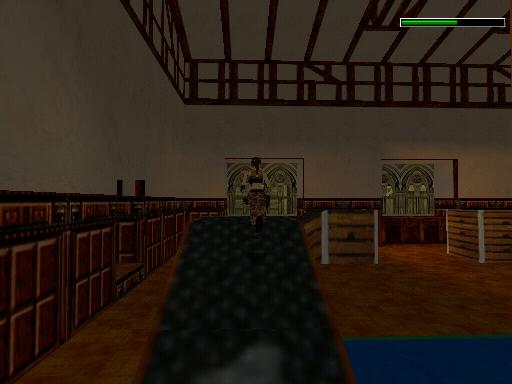The image showcases a scene from a video game. In the top right corner, there are green bars that add a touch of color contrast against a darker background. The top perimeter of the image features a wooden frame that encases the scene, complemented by white walls that offer a clean backdrop. To the left, red tiles can be seen, forming a continuous pathway that leads around the foreground of the image. Central to the scene is a carpeted ramp that ascends to a raised platform, which is supported by sturdy wooden boards and white structural supports. This elevated area overlooks a gap that players must jump across to reach the next platform. The primary floor area of the image is predominantly brown, adding a grounded and earthy tone to the overall setting.